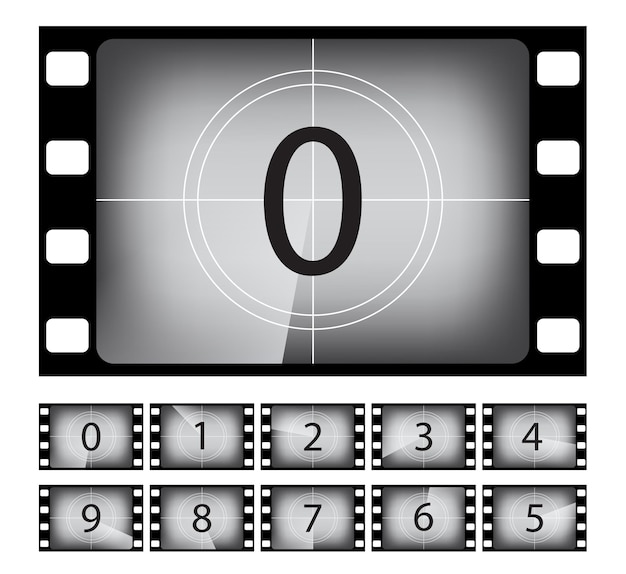This image depicts a black-and-white graphic that resembles an old-time movie editing tool. Central to the graphic is a large depiction of a film frame with the number "0" prominently displayed within a gray background and dissected by both vertical and horizontal lines. Below this main frame, there is a sequence of numbers from 1 to 9, each within its own smaller film frame. These frames, all resembling old-timey movie reels, have small white squares on their sides set against a black background, giving the impression of film perforations. The design evokes the count-down sequence traditionally used in film editing to mark the start of a reel, highlighting the transition through numbers that typically begin from 9 and proceed to 0, creating a full-circle effect. This detailed portrayal of countdown leader film is intended for editors or directors to use in synchronizing and editing film sequences.